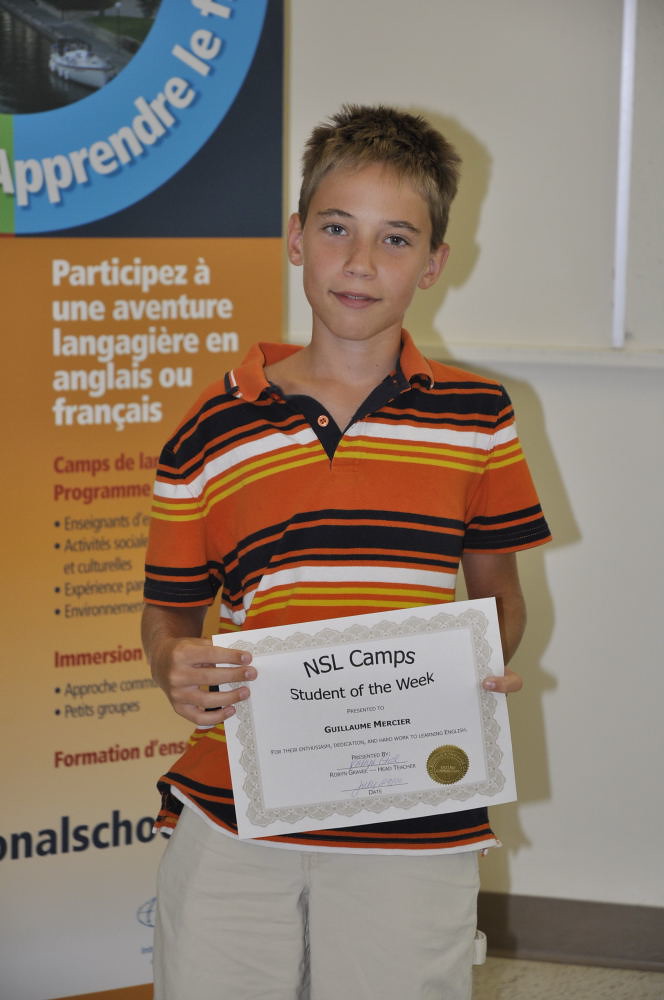This is a photo of a young boy named Jean Messier, estimated to be between 10 and 13 years old. Jean, who has short, sandy blond hair that's styled in a slightly spiked-out manner, is holding a certificate in front of him with both hands. The certificate, adorned with a decorative border and a gold seal on the lower right, reads "NSL Camp Student of the Week," along with Jean's name and a signature. Jean is dressed in a horizontally striped polo shirt featuring black, yellow, white, and orange colors, paired with khaki shorts or pants. Behind him stands a tall billboard sign with text in Spanish, translating to "participate in a language adventure in English or French," indicating the bilingual nature of the NSL program. The background includes an off-white wall and a darker brown running board on the right. Jean is facing the camera with a neutral expression, not quite smiling.